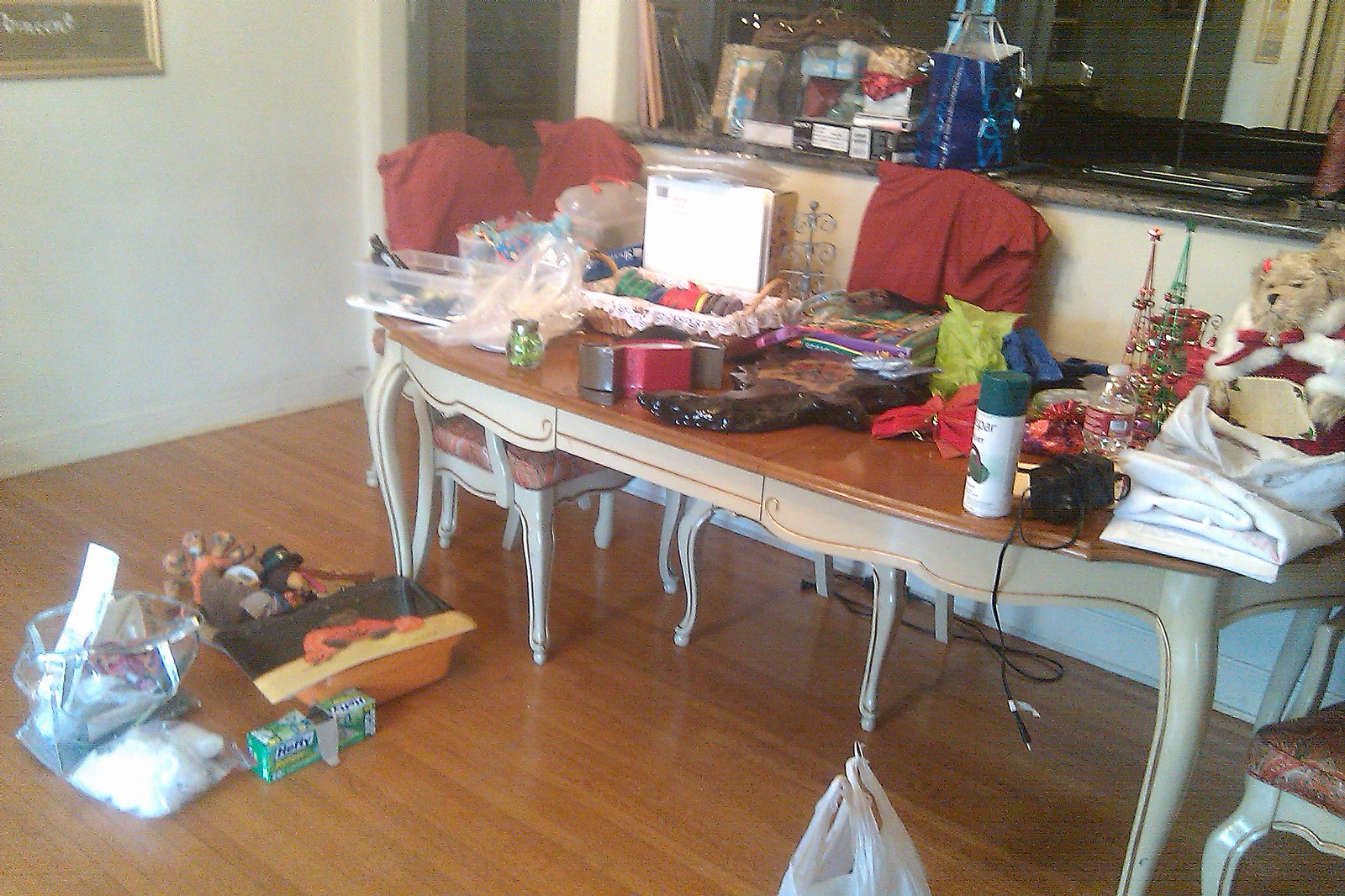The image depicts a dining area seamlessly connected to a kitchen. At the center of the room stands a long, antique dining table set, featuring a light brown tabletop and intricately designed ivory-colored sides with scalloped edges. The table rests on elegantly rounded legs adorned with golden pinstriping and a graceful curve in the middle. The table itself is cluttered with various items, including metal Christmas tree decorations, a bear figurine dressed in a red coat with white accents, a red bow, a can of spray paint with a green lid, multiple bows, a charger, and an assortment of craft materials, giving the impression of an ongoing project or activity.

Matching the table, the chairs feature red fabric seating and backs, complementing the festive theme. On the floor nearby, there is a box of Hefty trash bags. In the background, a stuffed turkey wearing a green hat adds a playful touch to the scene, contributing to the overall holiday vibe.